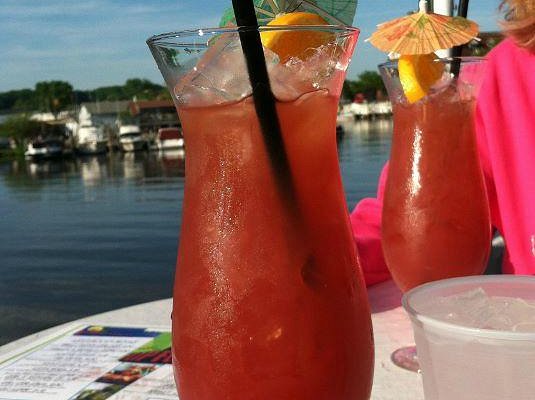This photograph captures a picturesque waterfront setting, likely at a beachside restaurant, given the presence of menus on the table. Central to the image are two vibrant, red cocktails served in tall, elegant hurricane glasses with bulbous bottoms that narrow and then flare out at the top. Each drink is festively garnished with a slice of orange, a green accent, a paper umbrella, and a straw. A glass of ice water is also visible in the foreground on the large, white table. The background reveals calm, rippling water, suggesting the scene is at a serene lake or harbor, with multiple boats and yachts docked across the shoreline. Adding a human element, part of a person in a bright pink shirt can be seen, likely preparing to enjoy one of the colorful drinks. The sky overhead hints at dusk, enhancing the tranquil and inviting atmosphere of the scene.